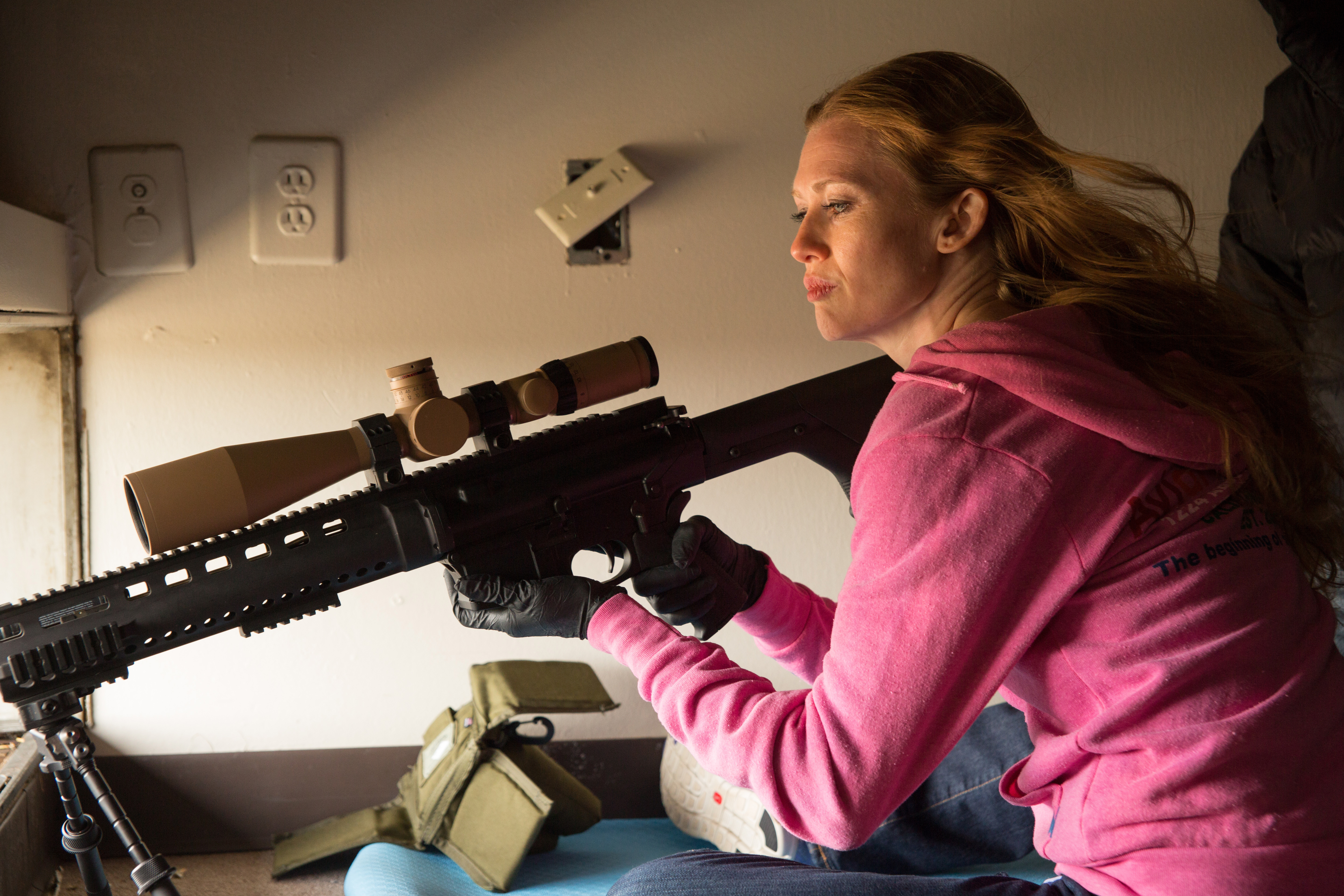In a scene reminiscent of a movie still, a woman with long, reddish-blonde hair and striking blue eyes is deeply focused as she prepares to shoot a black sniper rifle equipped with a large tan scope. Dressed in a pink hoodie with some lettering on the back and a pair of jeans, she ensures her aim by stabilizing the weapon on a tripod and carefully holding the shooting mechanism with both hands, which are covered in black leather gloves. The rifle is positioned to shoot out of a window, indicated by the light filtering in. Around her, the room appears disheveled; the beige wall behind her has multiple electrical outlets, one of which is hanging loosely with its faceplate askew. A blue rug lies partially on the floor, and a tan, open box likely for ammo sits nearby. Her concentration is evident, with her lips pursed and eye intently gazing through the scope. The sole of her right shoe, white and clean, angles into view, juxtaposing the room's cluttered state.